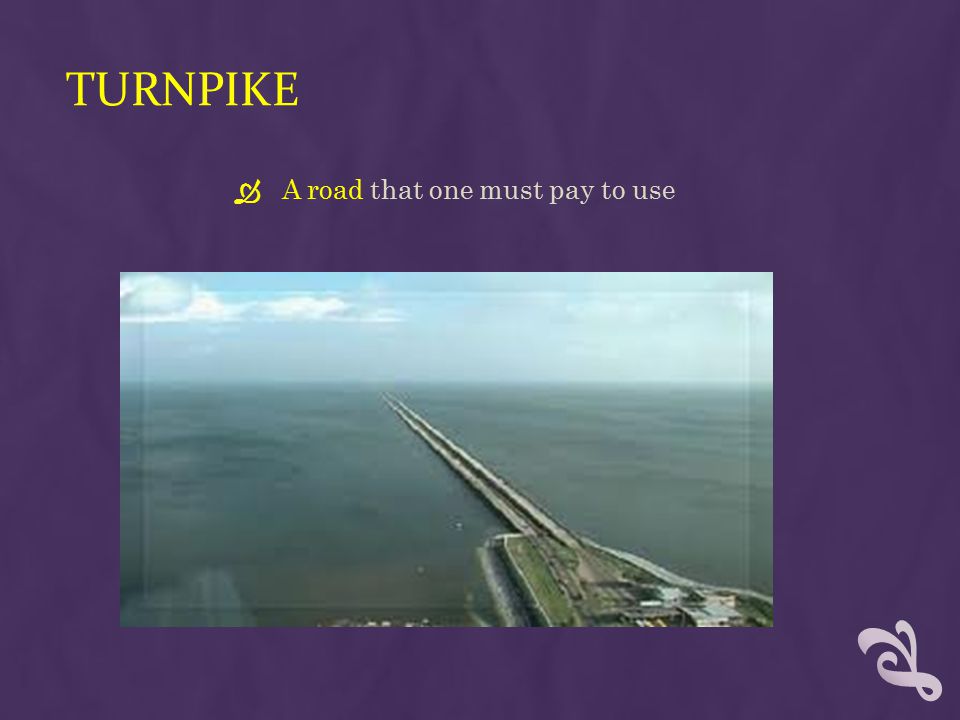The image features a digital, textured purple backdrop with faint white swirls, giving it a smoky appearance. In the upper left corner, the word "Turnpike" is prominently displayed in large yellow capital letters. Just below it, staggered more toward the center, are the words "A Road" in yellow, followed by "that one must pay to use" in a very light purple color. Centered against this background is a photograph that appears somewhat blurry. The photo depicts a long, imaginary road extending from a patch of grass and possibly a small city, over a vast expanse of ocean, disappearing into the horizon. The background of the photo transitions from blue and white sky with gray clouds to gray ocean water, suggesting a bridge-like structure disappearing into the distance. In the bottom right corner of the image, there is a white cursive symbol. The overall composition might symbolize the arduous, seemingly endless journey toward success.